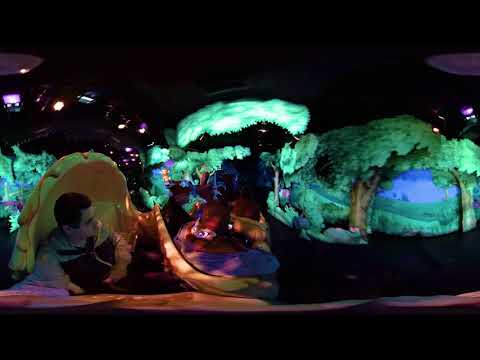The image is very dark and blurred with a multitude of colors making it hard to discern details clearly. On the left side, a man with dark hair, his face looking to the right, is partially visible along with his chest and hands. He appears to be sitting or leaning in a yellow plastic pod or sculpted enclosure that has a shell or cone shape. His legs are not visible. Overhead lights illuminate parts of the scene. Behind the man, there are vivid green, cartoony trees and blue sky, suggesting a constructed indoor wooded area. This area could be part of a themed amusement park ride, such as those found at Disney World. The whole scene is framed in darkness, with the right side of the photo showing more green trees, possibly fake, against a dark background. The green area in the center adds a cloud-like illusion over this dark region with faint images of foliage and water. The overall setting combines indoor stage lighting with vibrant colors, giving it a psychedelic or staged appearance. The obscure, dark mood suggests it might be a float in a nighttime parade or a dark ride attraction.